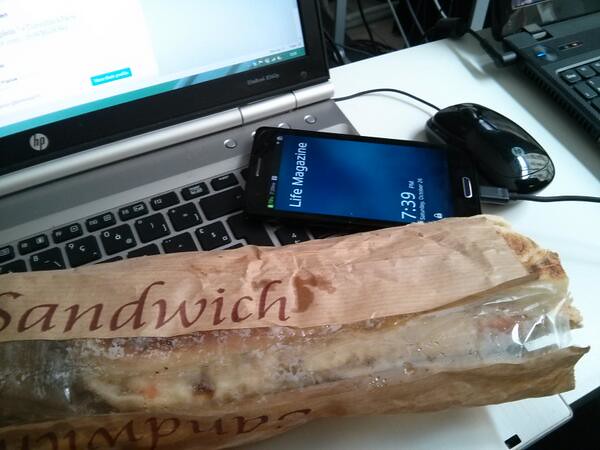The image depicts a cluttered indoor workspace centered around a white desk. Positioned primarily in the middle of the image is an open silver HP laptop with a long, partially eaten sub-sandwich sitting directly on its keyboard. The sandwich is wrapped in a bag that appears slightly wet with condensation, and the wrapper is labeled "sandwich." Next to the sandwich on the keyboard is a black Android smartphone displaying the "Life Magazine" cover and the time, 7:39 PM. The phone is plugged in and charging. Adjacent to the phone is a wired black computer mouse. In the upper left corner, we can see part of another white table with a second, partially cut-off black laptop that is also connected to various cords. The background features additional cables and peripherals, reinforcing the indoor setting of what appears to be a computer room. The visible colors in the image include white, green, blue, black, gray, brown, tan, and dark blue.